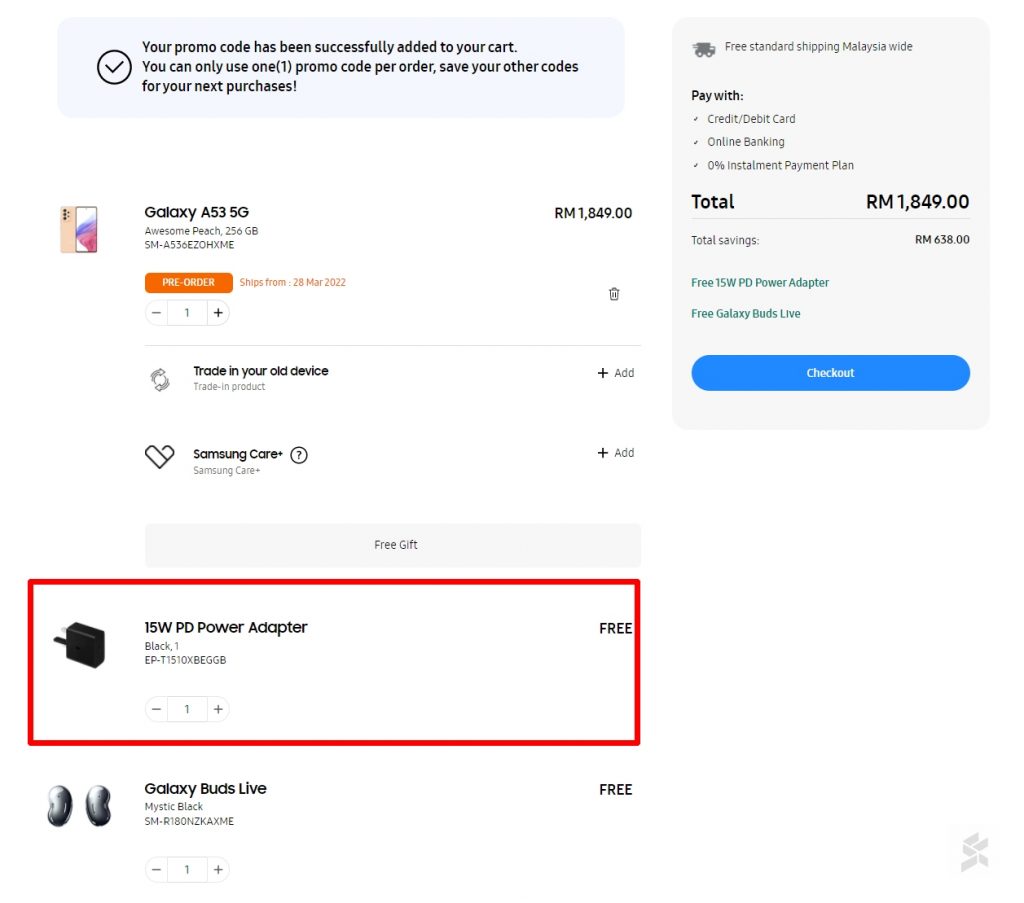**Detailed Product Page Description:**

The product page displays a variety of details and interactive elements for the Samsung Galaxy A53 5G. 

1. **Notification Box (Top Left)**:
   - A notification box is prominently displayed at the top left of the page. It features a check mark in black, accompanied by a message stating that the promo code was not successfully added to the cart. The message further explains that only one promo code can be used per order, advising customers to save other codes for future purchases. 

2. **Product Information**:
   - **Product Name:** Galaxy A53 5G
   - **Color:** Awesome Peach
   - **Storage Capacity:** 236GB
   - **Model Number:** SMA530EZ0HXME
   - **Price:** RM1849

3. **Pre-Order Button**:
   - An orange pre-order button indicates that the product is available for pre-order and will ship from March 28, 2022. 

4. **Icons and Widgets**:
   - **Trash Can Icon:** Located nearby, likely to remove items from the cart.
   - **Quantity Widget:** Displays the selected quantity with a horizontal gray line underneath.
   - **Trade-In Option:** An option to trade in your old device is mentioned with a plus sign to add details.
   - **Samsung Care Plus:** Accompanied by a question mark, potentially linking to more information about the protection plan.
   - **Free Gift Icon:** Denoted by a gray icon, indicating the availability of a complimentary item.

5. **Promotions and Free Gifts**:
    - A red box is superimposed around the product description, highlighting the offer of a free 15W PD power adapter.
   - The product page states that the Galaxy Buds Live are also included as a free gift, presented in black text with an icon to the left.

These elements combine to create a detailed and comprehensive overview of the product, its price, available promotions, and additional services.